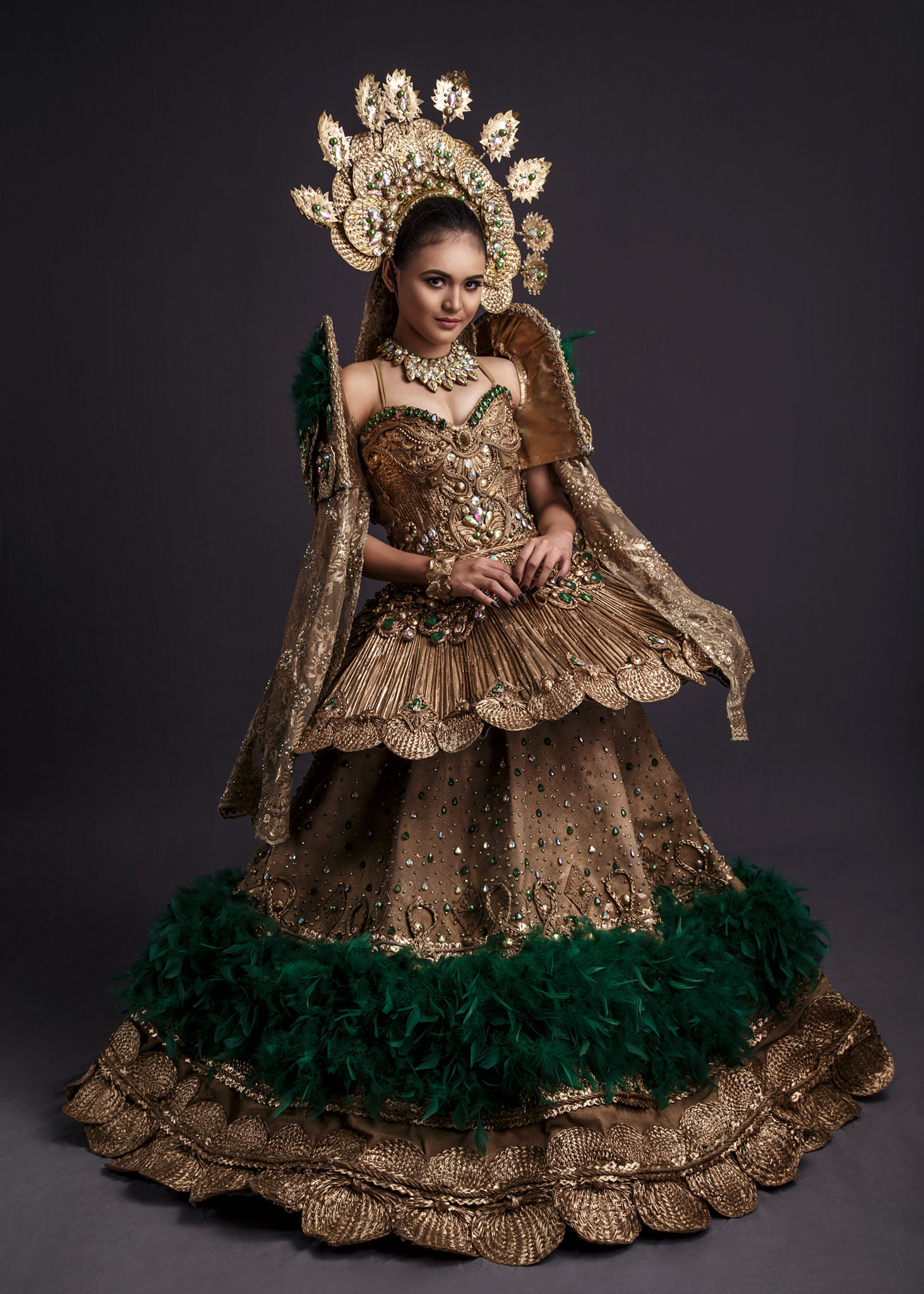This image features a young Asian woman dressed in an elaborate and intricately designed formal costume. The centerpiece of her attire is a gold floor-length dress, adorned with ornate designs and detailed craftsmanship. Around the lower portion of the dress, just above the bottom edge, is a band of green feathers, adding a textured contrast to the golden fabric. The upper part of the dress includes an ornate torso piece with delicate shoulder straps and intricate decorations. Her mid-section and breast area are accentuated with intricate patterns and a rim of green jewels. Draped over her shoulders is a shawl-like accessory that complements the overall opulence of the outfit.

Enhancing her regal appearance, the woman dons a large, golden headdress that resembles a fan, intricately designed with protruding golden elements. Her accessories include a thick, elaborate necklace adorned with multiple jewels and a pair of golden bracelets that accentuate her wrists. The photograph is taken against a dark gray and black background, which makes the colors of her attire—gold, green, and hints of gray—stand out vividly. The image is clear and professional, with the woman posing directly towards the camera, highlighting the exquisite details of her costume.